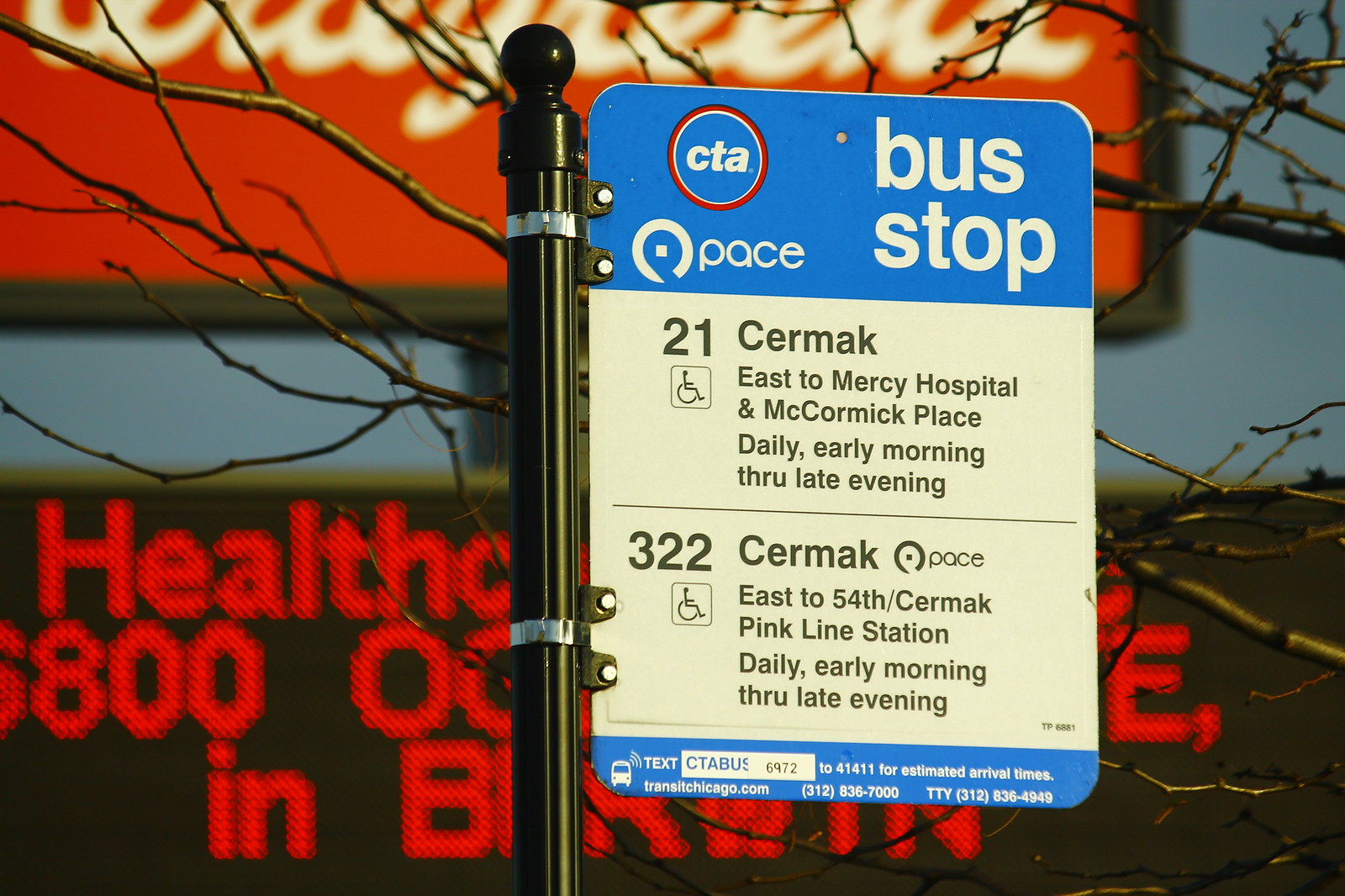In the foreground of the photograph stands a bus stop sign mounted on a sleek black metal pole with a rounded ball top. The sign, affixed to the pole with two steel bands, features a rectangular shape with rounded edges. The top section of the sign is a vivid blue background displaying a red circle with the white letters 'CTA' inside, alongside a smaller white circle with the 'Pace' logo. To the right of these symbols, the phrase "Bus Stop" is printed in bold white letters. Following this, the sign provides route details: 

- Route 21 Cermak, East to Mercy Hospital and McCormick Place, operating daily from early morning through late evening, with a handicap symbol beside this information.
- Below that, Route 322 Cermak Pace, East to 54th Cermak Pink Line Station, also running daily from early morning to late evening, accompanied by another handicap symbol. 

Further down, there are additional details including a number to text for estimated arrival times, a website (transitchicago.com), a contact number, and a TTY number. 

In the background, a red and white Walgreens marquee with a black border is visible, though partially obstructed by the sign. Below this marquee, there is another digital display with red text, difficult to read due to the interference from the bus stop sign. Tree limbs frame the scene, extending into the image from both the left and right sides.